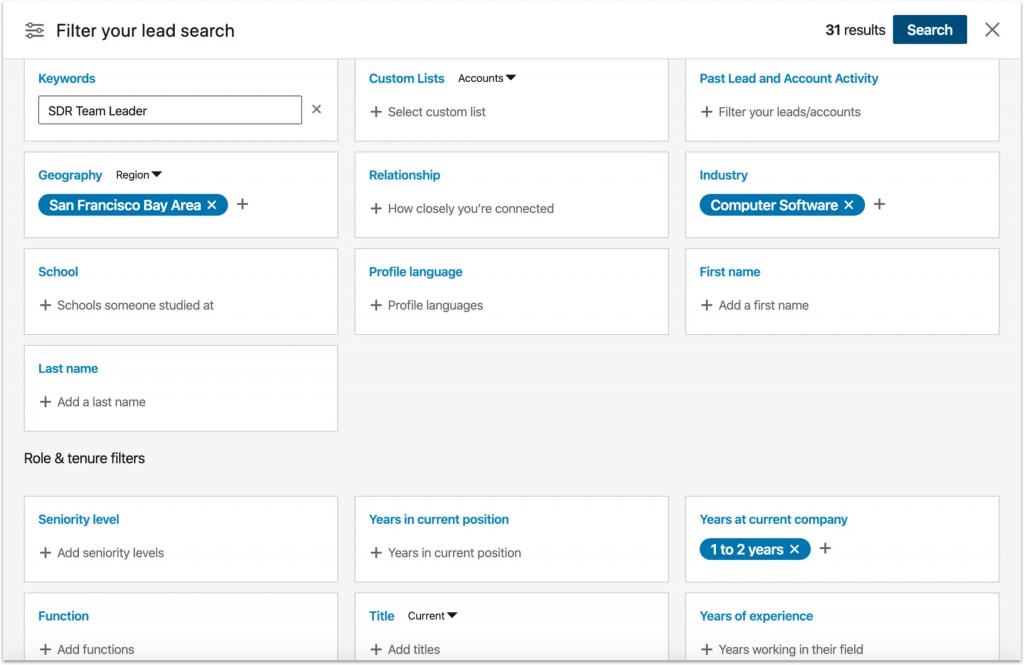This image, titled "Filter Your Lead Search," prominently displays its name in the top-left corner. On the opposite side, in the top-right corner, it states "31 Results" and features a search button accompanied by an 'X' icon, which allows users to cancel the action.

Below this section, the screen is populated with a series of white panels, each adorned with a blue heading. The first panel is labeled "Keywords," containing the text "SDR team leader" input by the user. The subsequent panel, titled "Geography," includes a dropdown menu set to "San Francisco Bay Area," with options to cancel or add values.

Following this are several more panels with additional filters:
- "School"
- "Last Name"
- "Custom Lists," which includes a dropdown for "Accounts"
- "Relationship"
- "Profile Language"
- "Past Lead and Account Activity"
- "Industry," currently displaying "Computer Software" with the option to change

Beneath these panels is a section labeled "Role and Tenure Filters," featuring more detailed filter options:
- "Seniority Level"
- "Function"
- "Years in Current Position"
- "Title"
- "Years at Current Company"
- "Years of Experience"

The image showcases a comprehensive lead search interface, complete with various parameters to refine and tailor the search results to specific needs.